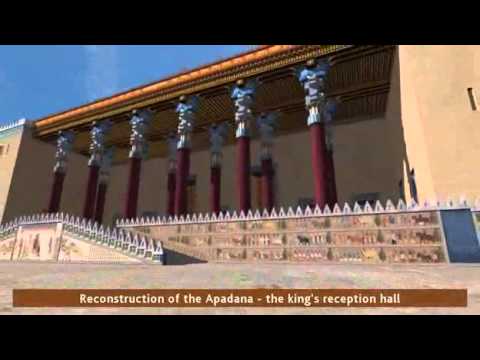The image depicts a reconstructed ancient building known as the Apadana, or The King's Reception Hall. The photo features a striking contrast between a vivid blue sky and the muted tones of the structure. Dominating the scene are six prominent burgundy columns with ornate silver tops and light blue accents. These columns are arranged in two rows leading toward a sandstone-colored courtyard. The foreground showcases a ramp or steps lined with silvery railings leading up to the elevated area of the hall. Below the columns is a long, decorated wall with fresco-like paintings. Just above the bottom black border of the image, there is a brown strip with white writing that reads, “Reconstruction of the Apadana – The King’s Reception Hall.” The structure includes a mix of colors—beige, light brown, dark brown, and blue—while the image is bordered by black bands at the top and bottom, making the light blue and silver details stand out against the darker hues.